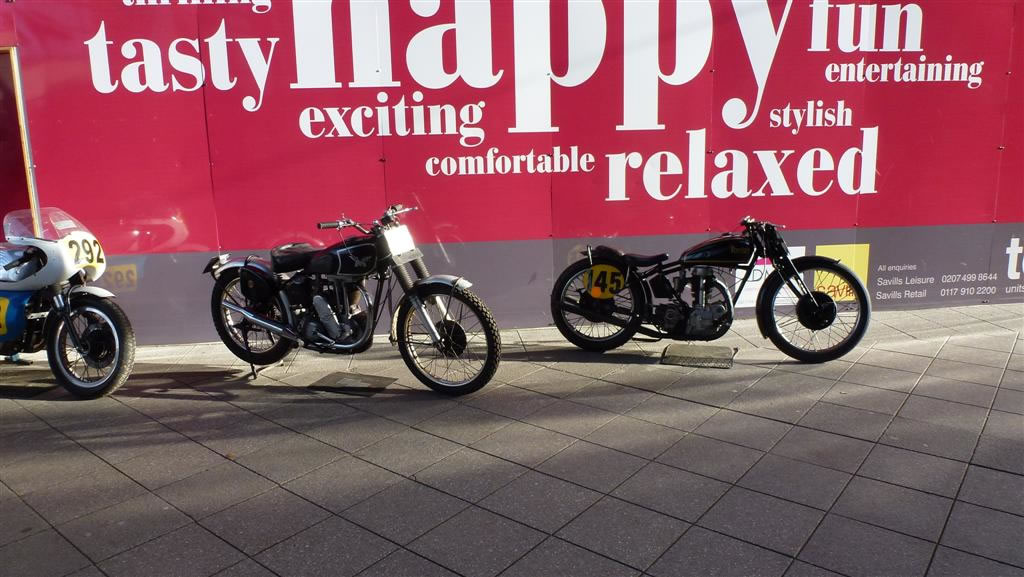In the image, three motorcycles are positioned on a square, gray stone pavement, appearing as black racing bikes. Each bike showcases distinct numbers: the leftmost bike is marked with the number 792, and the rightmost, featuring a sleek, aerodynamic design, displays the number 45 on its rear tire. A prominent red sign with prominently large, white letters serves as the backdrop, featuring the words "TASTY," "HAPPY," "FUN," with smaller accompanying text including "EXCITING" beneath "HAPPY," "ENTERTAINING" beneath "FUN," "STYLISH" beneath the "Y" in "HAPPY," "COMFORTABLE" beneath the "P," and "RELAXED" in larger letters to the right. The scene suggests an outdoor display, with the varying sizes of the words on the red sign creating a visually engaging backdrop for the similar structured motorcycles.